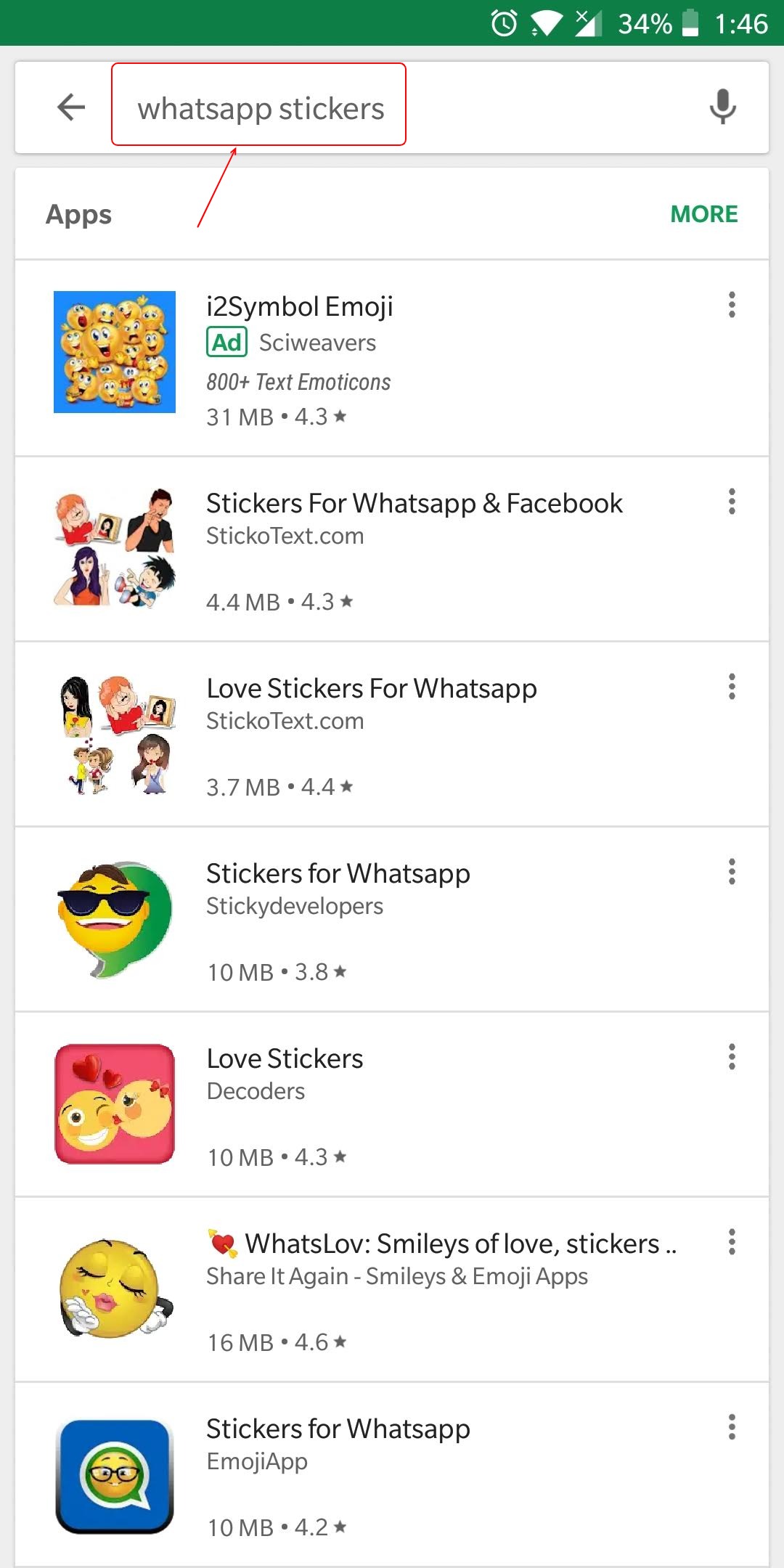The image displays a mobile phone interface with various elements related to WhatsApp stickers and other emoji applications. At the top, there's a long green rectangle, with a battery indicator showing 34% on the right and the time listed as 1:46. 

A red square outlines an area labeled "WhatsApp Stickers," with a red line extending downward from its bottom middle. To the left of this, the word "Apps" is displayed. 

Below, there's a blue square filled with at least 20 yellow emoji faces, characterized by large eyes and expressive mouths. Beside this, the text "I ❤️🛒 Add" appears. 

Further down, the header "Stickers for WhatsApp and Facebook" is accompanied by animated images of people on its left. Below, the section titled "Love Stickers for WhatsApp" features similar animated characters. 

Next, under the heading "Stickers for WhatsApp," there's an emoji with sunglasses and a green circle background. Below this, the caption "Love Stickers" appears, showcasing an emoji kissing another with red hearts as the background. 

Continuing, the section "What's Love: Smileys of Love Stickers" displays an emoji with large red lips and eyelashes. Finally, inside a blue square at the bottom, a yellow emoji with glasses is shown, accompanied by the text "Stickers for WhatsApp."